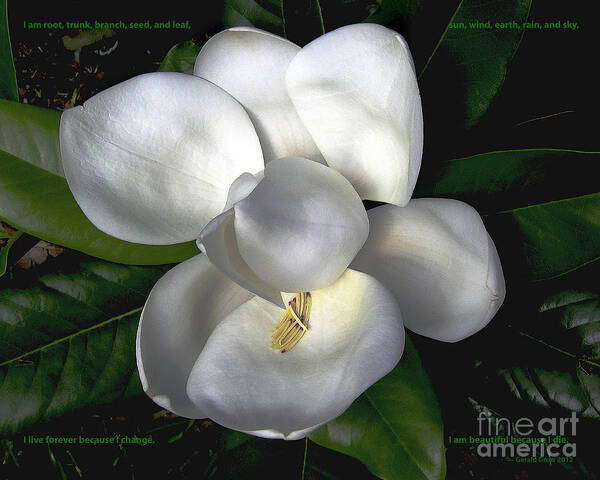This is a very detailed, close-up photograph of an exquisite white flower with three petals at the top and three at the bottom, meticulously resting atop vibrant green leaves. The white petals are centered and appear to have some gold pollen, suggesting a natural setting, despite an organized arrangement that might hint at artistic manipulation. Green text in the upper left corner reads, "I am root, trunk, branch, seed, and leaf," while the upper right corner states, "Sun, wind, earth, rain, and sky." In the bottom left corner are the words, "I live forever because I change," while the phrase, "I am beautiful because I die," appears in green text in the lower right corner, alongside a more prominent gray text reading, "Fine Art America." The photograph, with different shades of green in the background, potentially taken in the wild or a garden, emphasizes the flower as the central object, blending elements of art and nature.